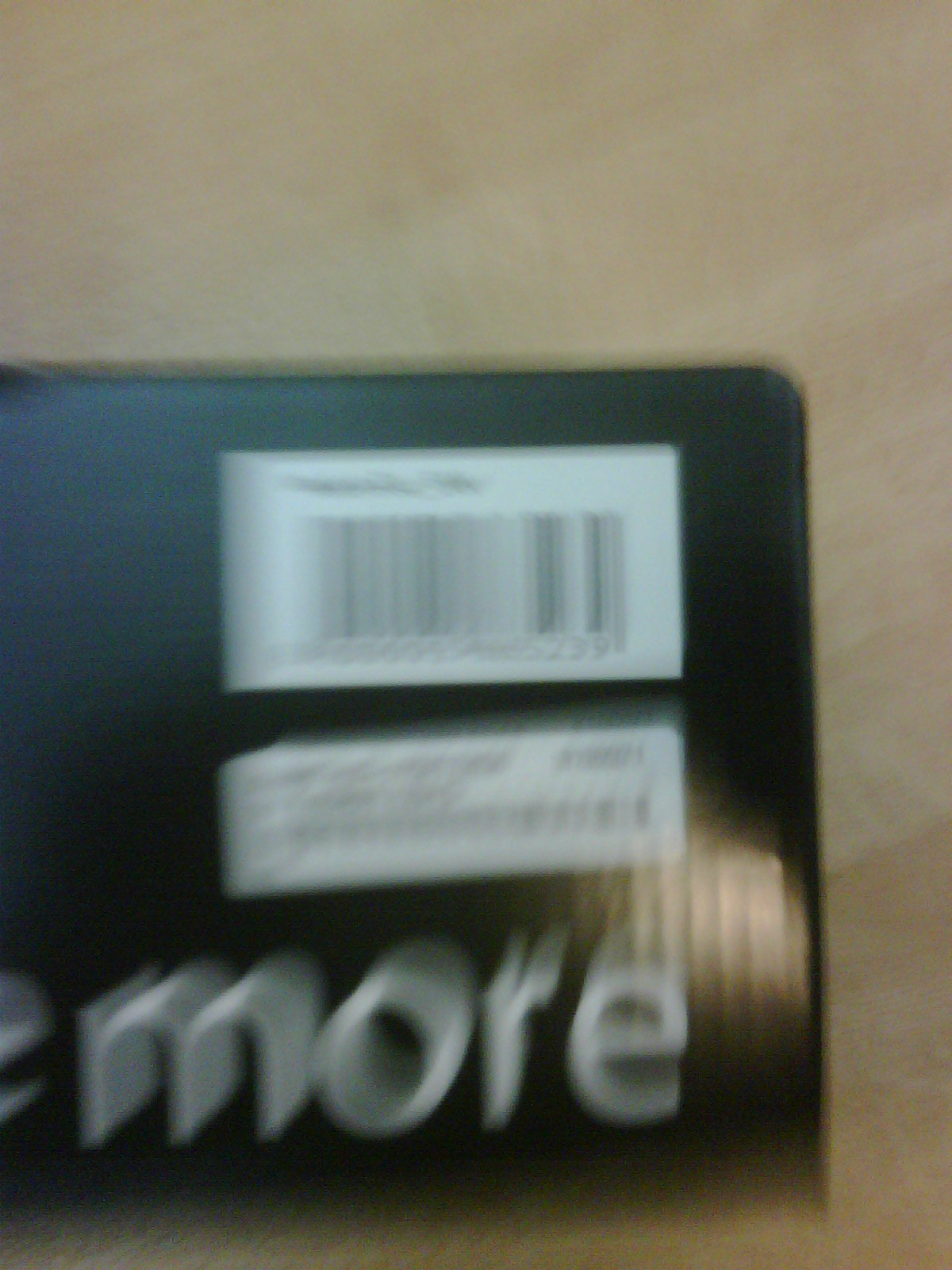The image depicts the top right corner of a box with a rounded edge. The box features a noticeable label for scanning, positioned on a white section, possibly used for checkout. Beneath this white area on the black surface of the box, there's a smaller, less discernible label, the purpose of which is unclear. Below the box, a smaller white box is present, showing some text that reads "more" in white letters, although the image's blurriness makes it difficult to read clearly. Light from an unknown source reflects off the box, and the entire scene is set against a light brown laminate floor.